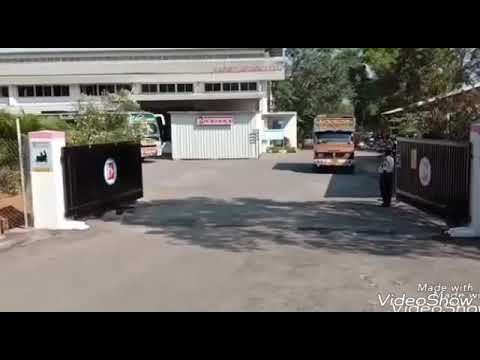The image captures the entrance to an important facility marked by large, fully-opened black gates flanked by tall white rectangular posts, some accented with a light pink color. A security guard stands on the right side of the gate, which opens inward, while another shadowed figure is discernible on the left. The facility appears to be bustling with activity: a weathered red pickup truck with a cargo storage on top is positioned towards the left, seemingly emerging from the gate. Adjacent to the truck, a large passenger van is visible in transit. The backdrop includes a long white building that resembles a small warehouse, devoid of windows on the lower part but featuring a row of windows above, running from the middle to the left edge, along with a metal corrugated steel booth near the bottom. Vegetation, including palm trees, adds a touch of greenery to the setting. Despite the low-resolution quality of the image and the unreadable signs, the scene clearly depicts a secure and significant establishment.